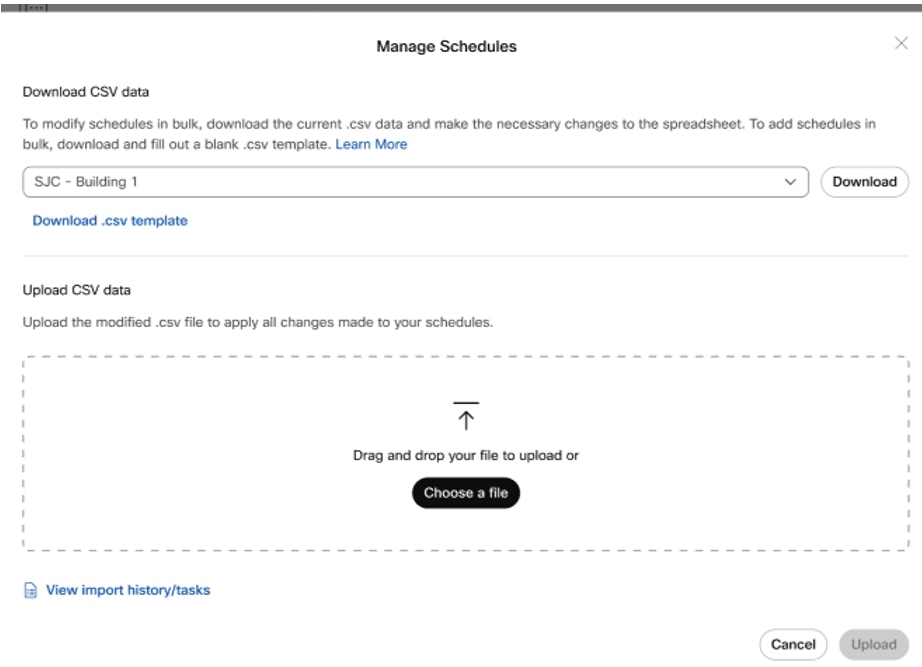A computer screen displaying a scheduling management interface is shown. 

At the top of the screen, there is a solid line running horizontally, followed by the header "Manage Schedules". Below this, there's an instruction section aiming to help users manage scheduling data. It includes options such as "Download CSV Data" and guidance text that reads: "To modify schedules in bulk, download the current .CSV data and make the necessary changes to the spreadsheet. To add schedules in bulk, download and fill out a blank .CSV template."

A clickable link labeled "Learn More" is highlighted in blue, suggesting additional resources or help.

Further down, a large rectangular box is labeled "SJC-Building1" with an associated button labeled "Download".

Below this box, another clickable link in blue text reads "Download .CSV Template". This is followed by a section titled "Upload CSV Data", instructing users to upload modified .CSV files to apply changes to their schedules. A dotted gray rectangle marks the upload area, indicating users to "Drag and drop your file to upload or choose a file," with "choose a file" presented in black text, emphasizing it as an actionable button.